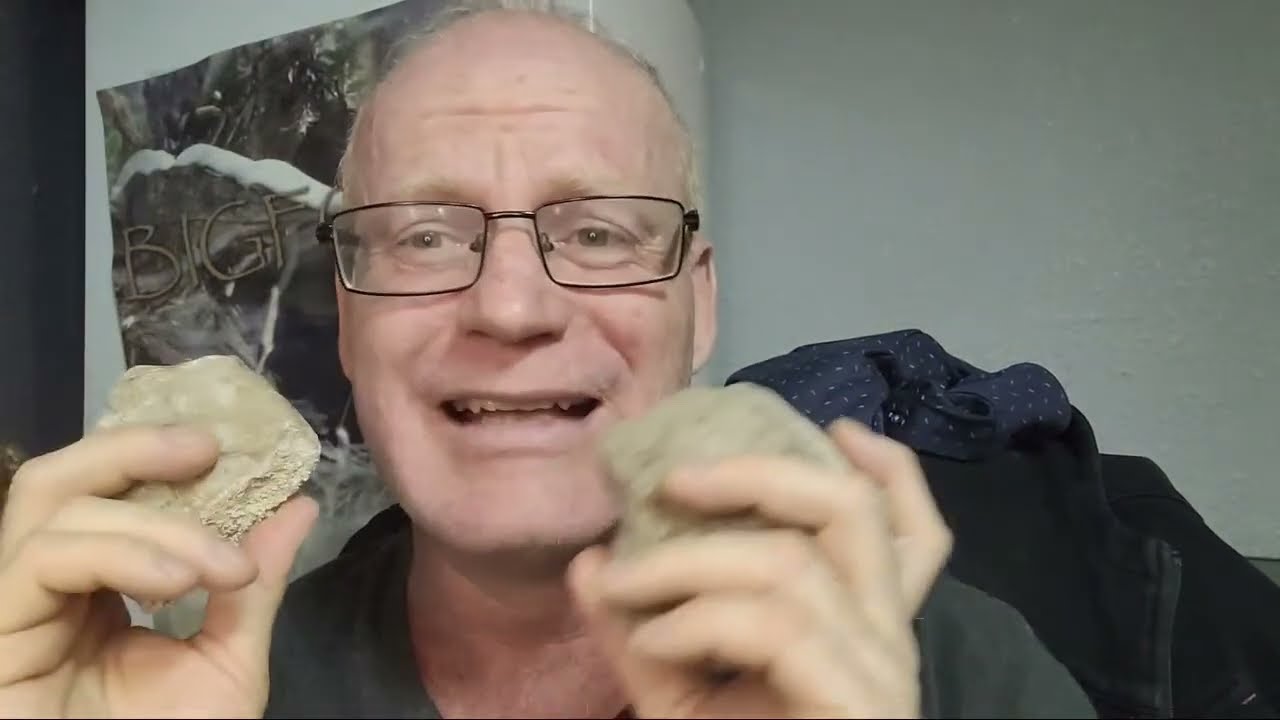This photograph features an older Caucasian male who is balding with sparse gray or blonde hair and wearing rectangular wire-rimmed glasses. He appears to be in the middle of speaking, with his mouth open and visible top and bottom teeth, looking slightly to our left, his right. He is holding up two tan, light-medium brown stones or possibly pieces of hard bread in both hands, which are slightly blurry due to their proximity to the camera. He is dressed in a gray T-shirt, with a black jacket draped over what seems to be a dark-colored chair behind him. The background consists of a white wall adorned with a black and white poster that partially reads "Big F" and possibly spells out "Bigfoot." The overall scene suggests he might be demonstrating or explaining something on video.